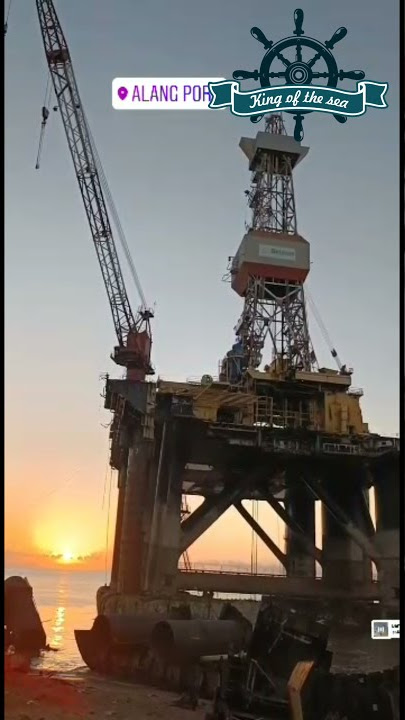The photograph features a massive offshore oil rig, possibly located in the Gulf of Mexico. The rig stands tall against a predominantly gray sky, colored with hues of orange and blue from an impending sunrise. Extensive steel beams and concrete pillars anchor the structure to the seafloor. Multiple layers and platforms are visible, along with yellow machinery and a large industrial crane extending out to the left side of the image. Superimposed text reads "Alang Por King of the Sea," with "King of the Sea" forming part of a logo that includes a traditional ship's wheel. The scene captures the sun's early light, enhancing the detailed industrial elements while casting a dim, dusky shade over the foreground. In the distance, the ocean is faintly visible, marking the horizon. Various bits of debris, including metal pipes, are scattered at the base of the oil rig.